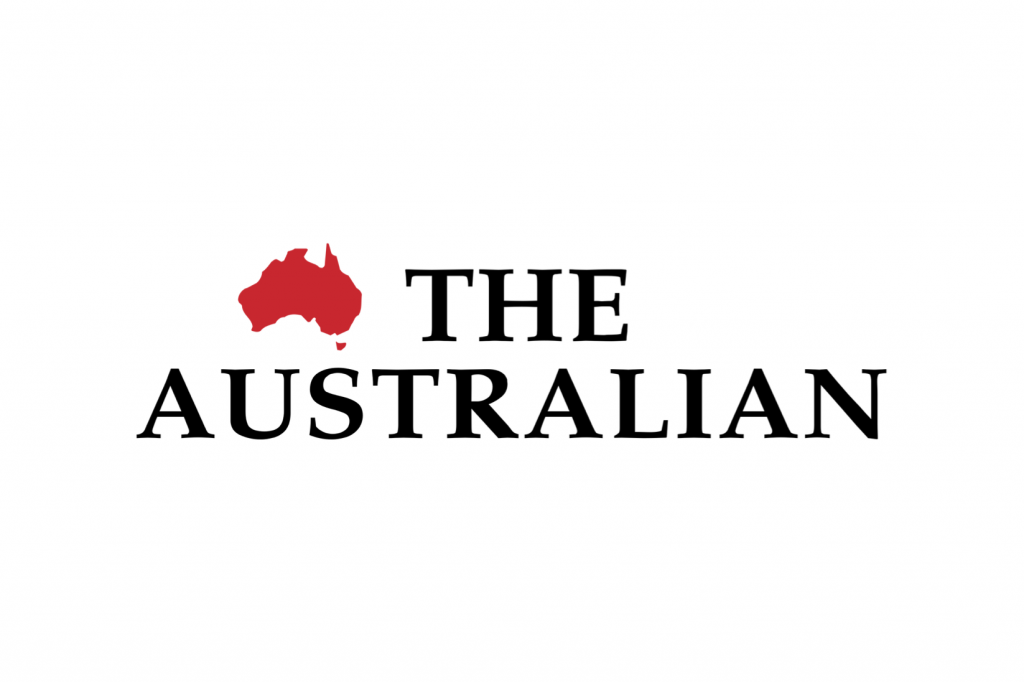The image is a rectangular graphic with a white background, oriented horizontally. Dominating the composition is a red silhouette of the continent of Australia, prominently displayed in the center. To the right of the red map, the word "THE" is boldly printed in large, capitalized black letters. Directly below "THE," the word "AUSTRALIAN" is also displayed in the same, capitalized black letters, making a clear and striking contrast against the pristine white backdrop. The overall design is minimalistic, featuring no additional elements or text beyond what is described.